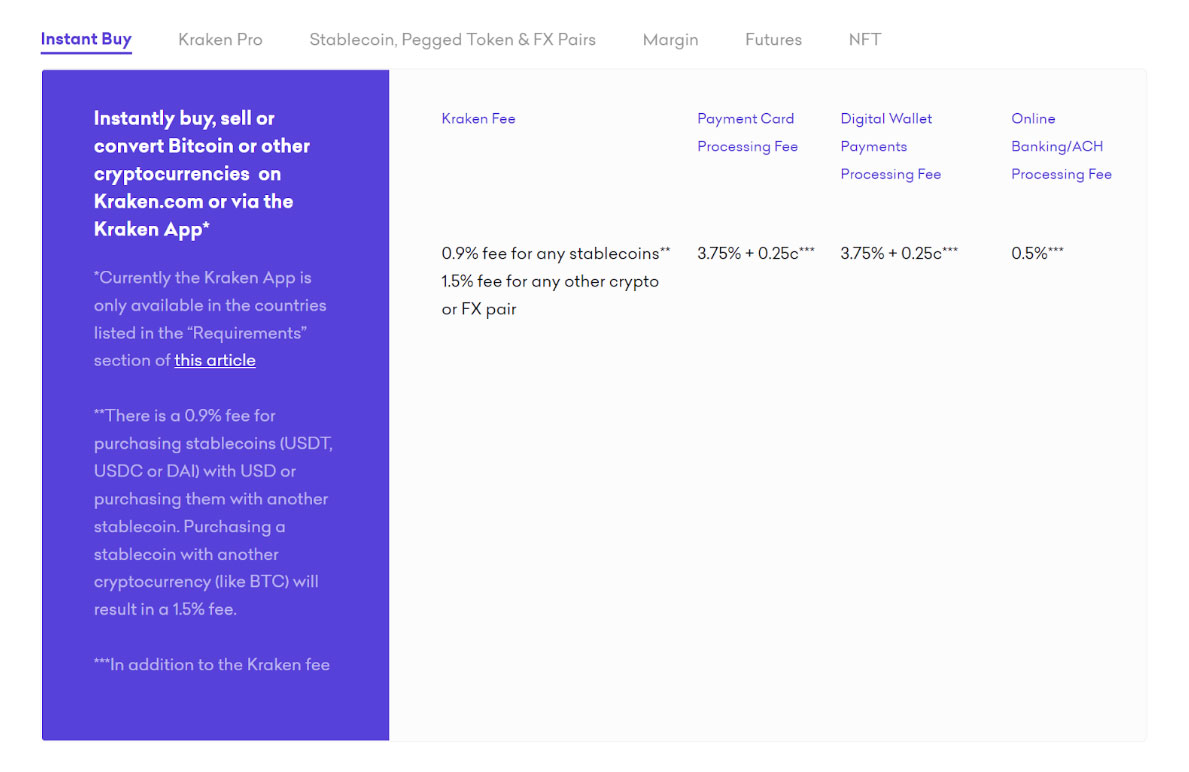On the Kraken.com website, the Bitcoin-related webpage features a clean, white background with a detailed and organized layout. Across the top menu bar, users can find various options including Instant Buy, Kraken Pro, Stablecoin, Peg Token, FX Pairs, Margin, Futures, and NFT. 

A striking, bright blue ribbon runs vertically down the left third of the page, catching the viewer's attention. At the very top of this ribbon, bold white text highlights the key functionality: "Instantly buy, sell, or convert Bitcoin or other cryptocurrencies on Kraken.com or via the Kraken app." Beneath this, in faint white text, there is a note: "Currently the Kraken app is only available in the countries listed in the requirements section of this article," linked by an embedded hyperlink.

Further down, the ribbon details the fee structure. There is a 0.9% fee for purchasing stablecoins such as USDT, USDC, or DAI with USD, or for purchasing them with another stablecoin. If a stablecoin is purchased using another cryptocurrency like BTC, the fee increases to 1.5%.

On the right side of the page, the top section outlines various fee categories: Kraken fee, payment card processing fee, digital wallet payments processing fee, and online banking ACH processing fee, ensuring that users are well-informed about the costs associated with their transactions.